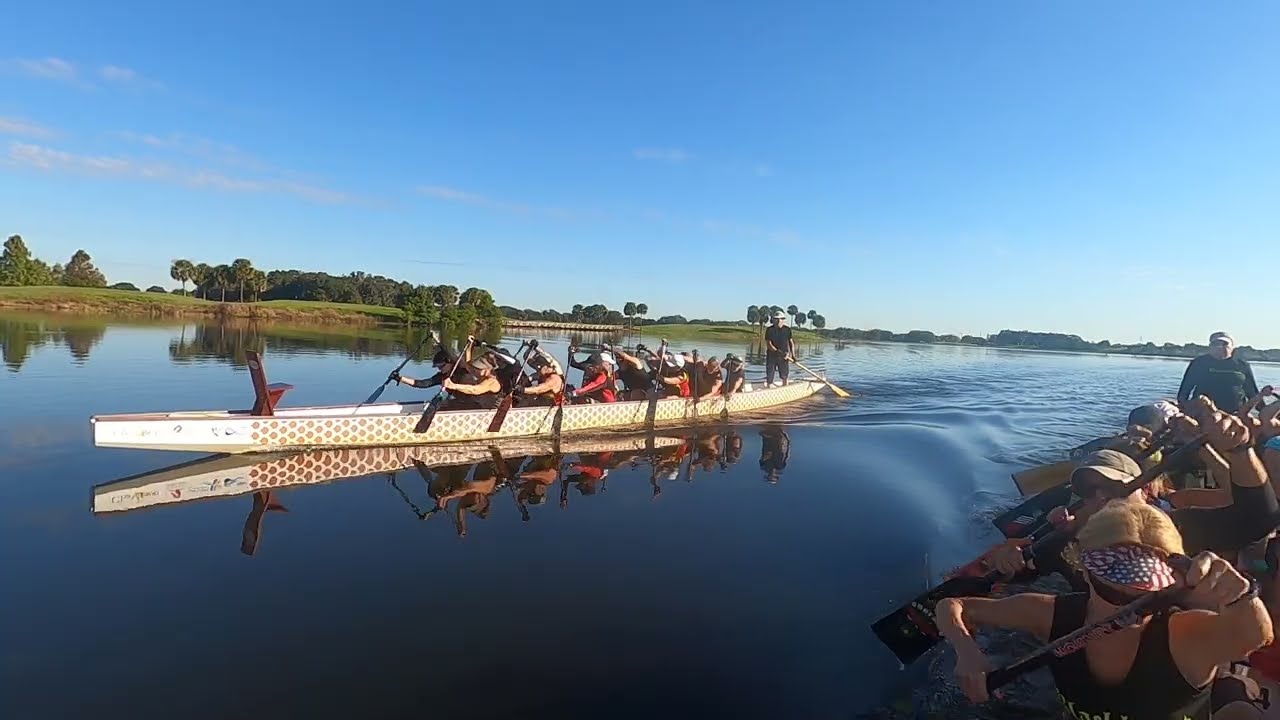The image captures a lively rowing scene on a large body of water, possibly a lake or river. Two long, canoe-like boats filled with dedicated and serious rowers dominate the scene, moving from the right side to the left side of the photograph, evidenced by the ripples in their wake. The boat on the left features a distinctive yellow and brown snakeskin or dragon scale pattern with a man standing at the back, possibly guiding the team, and an empty chair. The second boat, partially obscured as the photographer appears to be on it, also has rowers holding their oars aloft and another standing guide. The tranquil water appears dark and smooth, with no visible splashes from the oars. The background reveals a lush green shoreline adorned with various trees and shrubbery, maybe even some palm trees, against a backdrop of rolling hills that resemble a golf course landscape. Overhead, a bright blue sky dappled with light clouds completes the serene environment. The colors in the image span a vibrant palette of red, white, blue, green, gray, black, and yellow, and the photograph, capturing this dynamic yet calm moment, does not appear to be professionally taken.